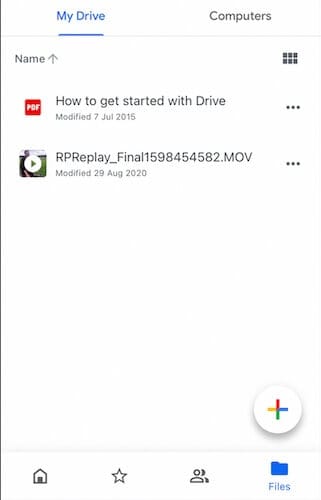This is a detailed caption for an image of a Google Drive interface captured on a phone:

---

The image displays a section of the Google Drive interface on a mobile device, set against a white background. On the left side, there is a prominent black vertical line. The top left features the text "My Drive" in blue font, with an underline in the same color. Adjacent to it, the word "Computers" is displayed in grey font, sitting above a thin grey line.

Further down on the left, the label "Name" appears in grey text accompanied by an upward-pointing grey arrow. Next to it, six small boxes are arranged in a single row. Below this, a red square with the white "PDF" logo is visible, followed by the text "How to Get Started with Drive" in black font. Directly beneath this, the date "Modified 7 July 2015" is displayed. To the right of this entry are three vertically aligned grey dots.

Below the first entry, another item is listed. On the left, there is a video thumbnail featuring a white circle with a grey triangle pointing to the right, alongside the filename "RPReplay_Final_1598454582.mov" in black text. Adjacent to this are three grey dots, and beneath the filename, the date "Modified 29 August 2020" is written. On the far right, there is a circular icon with segments colored red, yellow, blue, and green.

A thin grey line spans the image underneath these entries. Further down, an icon strip is displayed from left to right featuring a grey house, a grey outlined star, a grey outlined person with a shadow, and blue outlined files with an additional blue file icon above it. Another faint grey line runs beneath these icons.

---

This caption provides a comprehensive description of the image with precise details about the visual elements and their arrangement.